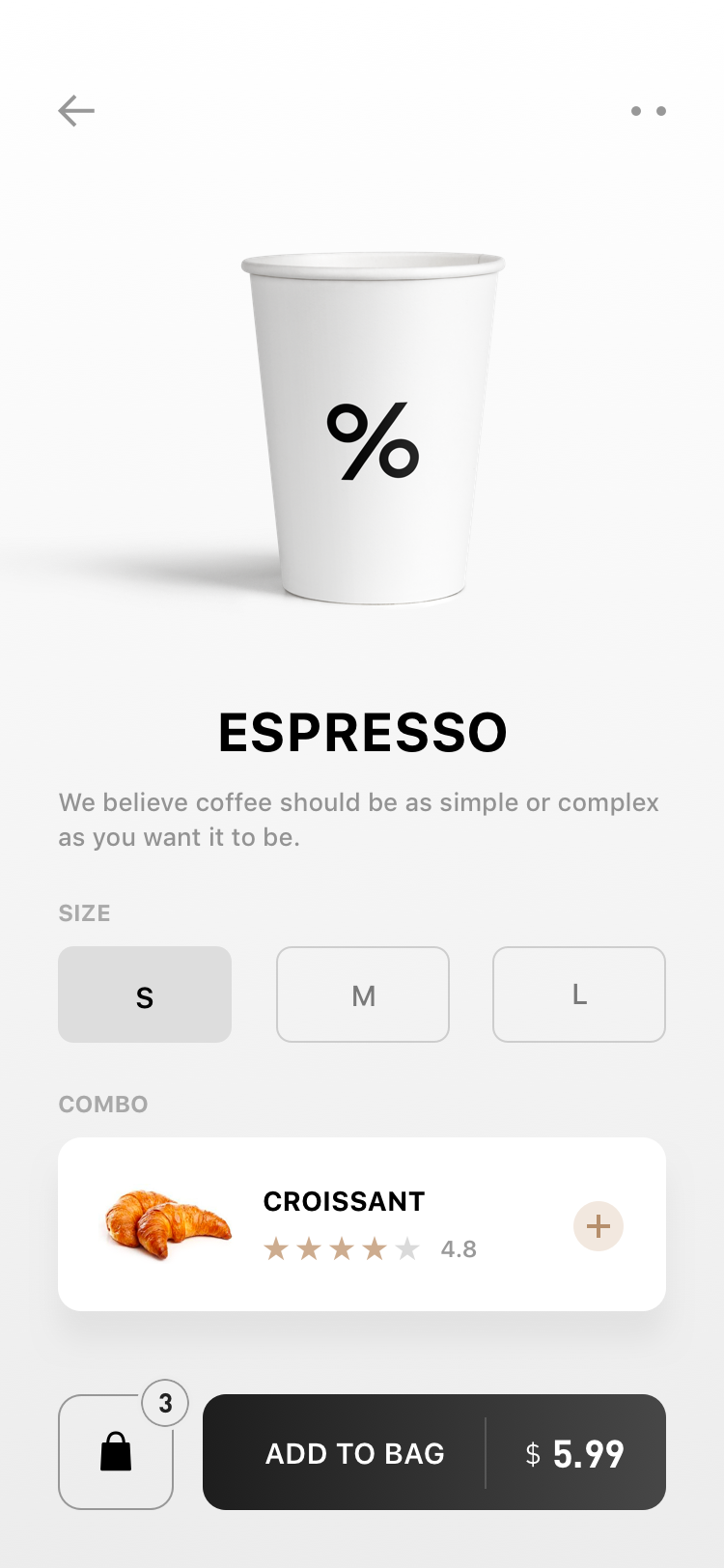The image showcases a mobile application for ordering coffee. The app is displayed on a phone with a clean, white background. At the top of the screen, an arrow is visible alongside two dots on the right-hand side. 

Central to the app interface is an illustration of a white coffee cup adorned with a black percentage symbol. Below the cup, the word "Espresso" is prominently displayed in bold, black letters. The tagline under the header reads, "We believe coffee should be as simple or complex as you want it to be."

Further down, the app offers size options for the coffee: small, medium, and large. The selected size is small, which is paired as a combo with a croissant. The combo has received a high rating of 4.8 stars. Additionally, there is a plus symbol to add more items to the order, depicted by a shopping bag icon that shows there are currently three items inside.

The "Add to Bag" button is prominently displayed in a black box with white text. The total cost at the bottom indicates $5.99, though it is unclear if this includes the croissant.